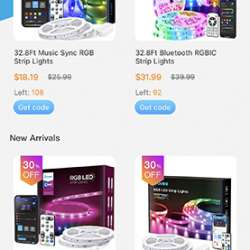The image appears to be a cropped screenshot of a product listing page, showcasing four items arranged in a two-by-two grid format. The top row of products is partially cropped out of view, leaving visible portions that resemble wheels or spools of LED strip lights. Specifically, the top left product is identifiable by its label, which reads "32.8 ft Music Sync RGB Strip Lights." Beneath this product title, the price is prominently displayed in orange text as $18.19. Adjacent to this, the original price of $25.95 is shown in gray and is crossed out, indicating a discount. Further down, the text "left: $1.08" is visible, likely referring to a remaining amount or a similar designation. At the very bottom of this product listing, a blue button labeled "Get Code" is available for interaction.